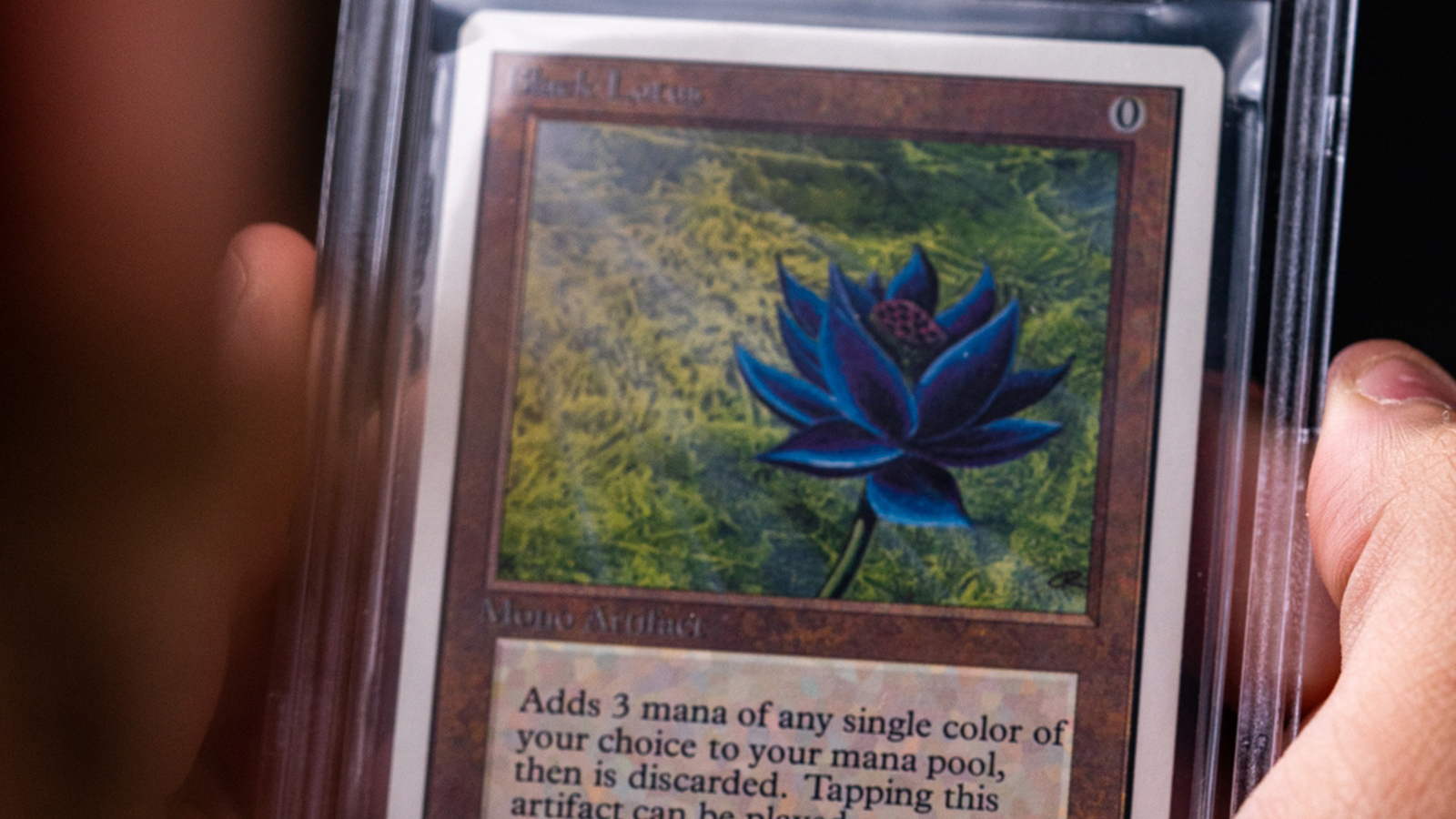The image depicts a close-up of a highly valuable "Black Lotus" trading card from the game Magic: The Gathering. The card, encased in a clear plastic protective case to preserve its condition, is being held by a hand, with the thumb and index finger visible. The artwork features a bluish-black lotus flower set against a grassy background. At the top left of the card, the name "Black Lotus" is displayed in black text, and at the top right is the number "0." The text box at the bottom left classifies it as a "Mono Artifact" and includes the partially visible description: "Adds 3 mana of any single color of your choice to your mana pool, then it's discarded." The remaining text is cut off by the photo, but it mentions that tapping this artifact results in further effects. The card is surrounded by a brown speckled background, enhancing its visual appeal and mystique.